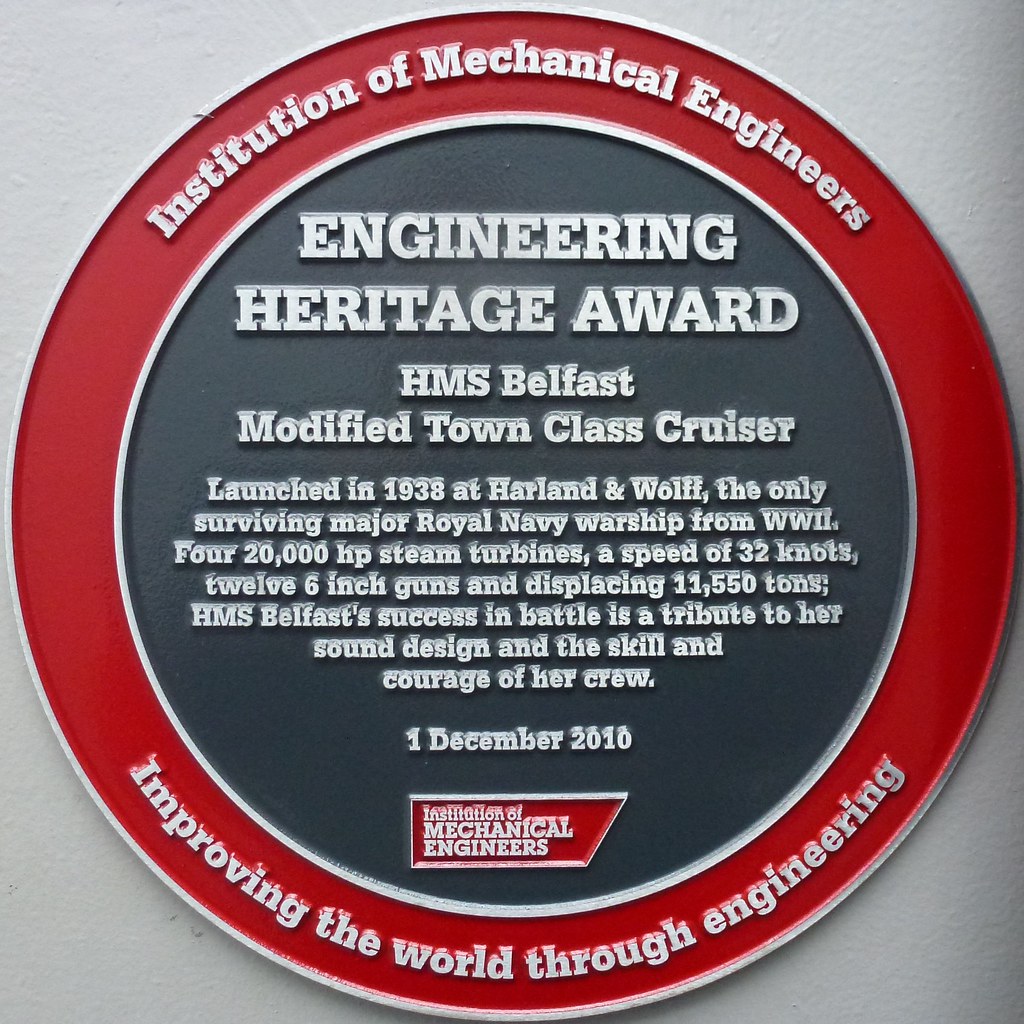This is a detailed description of an award plaque from the Institution of Mechanical Engineers, prominently featuring the text "Improving the World Through Engineering" around its outer red circle, with a gray center and white font. The plaque, dedicated on December 1, 2010, commemorates the HMS Belfast, a Modified Town Class Cruiser. Launched in 1938 at Harland and Wolff, the HMS Belfast is celebrated as the only surviving major Royal Navy warship from World War II. The plaque highlights the ship's impressive specifications: 20,000 horsepower steam turbines, a speed of 32 knots, armament of twelve 6-inch guns, and a displacement of 11,550 tons. It attributes the ship’s success in battle to her sound design and the skill and courage of her crew. The elegant and clean design of the plaque suggests it could serve as an outdoor heritage sign.